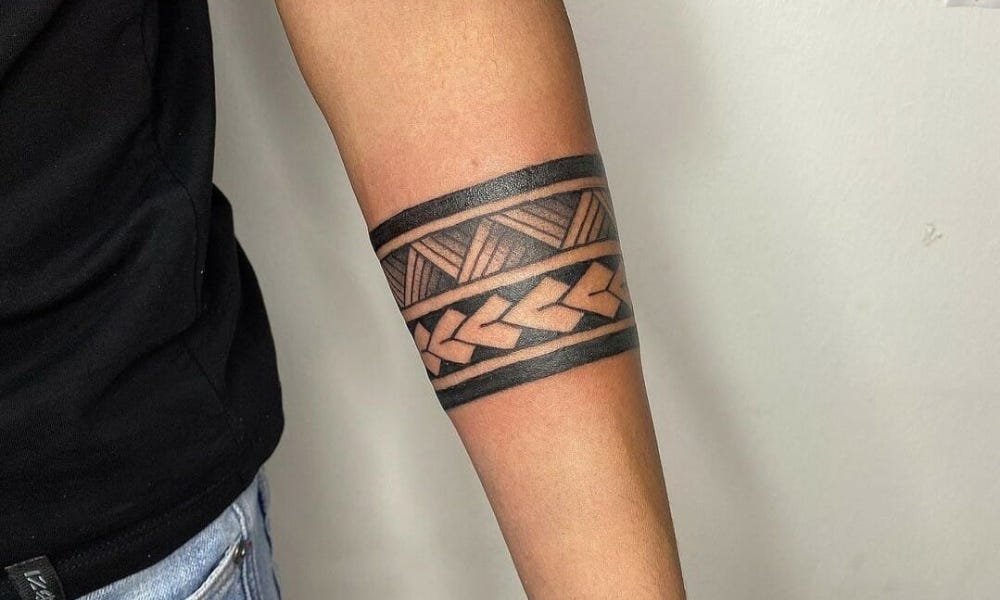The image depicts a person's forearm adorned with a detailed tribal band tattoo, distinctly styled in an indigenous manner. The tattoo, approximately three to four inches in width, features a striking contrast of black ink and the person’s fair, slightly tanned skin. The design is elaborately segmented: the top starts with a thick black line, followed by a skin-toned band, then a series of shaded, 3D-like triangles pointing in opposite directions. Underneath this section is another narrow skin line. The lower part of the tattoo showcases a black background with horizontally oriented, skin-colored heart shapes outlined in black, creating a visual impression reminiscent of stylized arrows. This band pattern is capped with another skin line and a thick black line at the bottom. The person is dressed in a black t-shirt and blue jeans, and is positioned against a white background, with the tattooed arm prominently displayed.